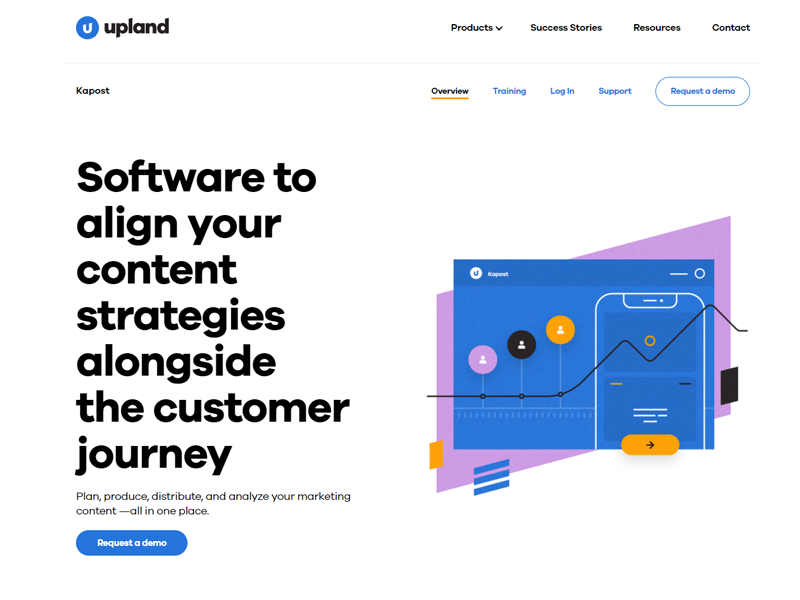The image depicts a startup website for a company named "Upland." In the upper left corner, there is a distinctive blue circular logo featuring a white "U" and the company name "Upland." To the right of the logo, there is a navigation menu with the sections labeled: "Products," "Success Stories," "Resources," and "Contact." 

Below this main menu, there are additional subsections listed as "Cut Posts," "Overview," "Training," "Login," "Support," and "Request a Demo."

The main focal point of the webpage is a large hero section that occupies a significant portion of the screen and is divided into two halves. On the left side, a prominent headline reads, "Software to align your content strategies alongside the customer journey." Below the headline, a subtext elaborates, "Plan, produce, distribute, and analyze your marketing content all in one place."

On the right side of the hero section, there is a mock-up diagram of a website, labeled "Composed," which appears to visually represent the layout and design of the actual application or service being offered.

At the bottom-left corner of this section, there is another "Request a Demo" button, distinguishable by its blue background and white text.

The overall design of the website features a predominantly white background, lending it a clean and modern aesthetic.